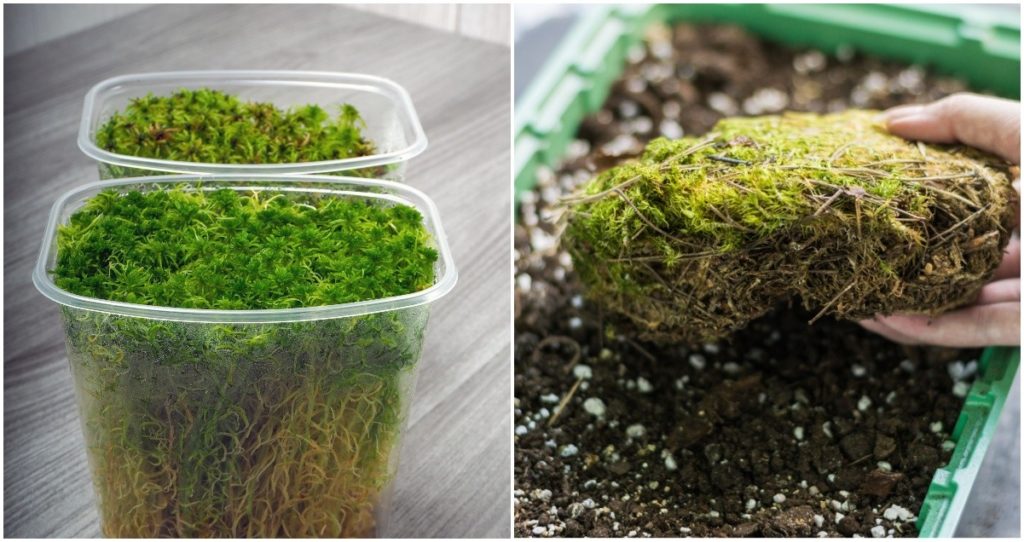This image is composed of two closely related photographs separated by a white vertical border. Each photo, occupying either side of the image, is of the same size and showcases different stages of plant growth involving sphagnum moss.

On the left side, two clear plastic containers sit side-by-side on a wooden table or counter. These containers, without lids, are filled with sphagnum moss, showcasing a gradient from lush green at the top to a yellowish hue towards the bottom. Condensation is visible on the inner sides of the containers, suggesting a humid environment ideal for the moss. The backdrop appears to be a gray street wall, contributing to the urban setting of the scene.

The right-side photograph features a green planting tray filled with dark potting soil, interspersed with white perlite chunks. A Caucasian hand, likely the right hand, is seen hovering over the tray, holding a sizable clump of sphagnum moss. The moss is vibrant green on top with visible root structures extending downward. The hand appears to be in the process of placing the moss into the soil, highlighting an active planting or propagation scene. The green tray is also set on a gray table, and the focus on the hand and the plant transitions into a slightly blurred background, emphasizing the subject in the foreground.